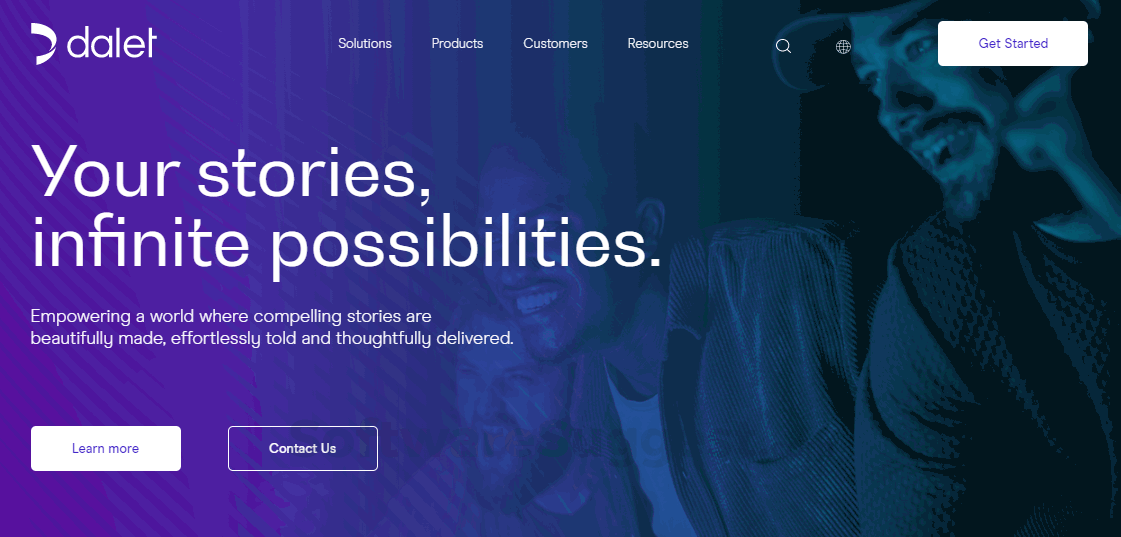The advertisement features a brochure for DALET, prominently displayed against a blue background. The scene includes three men engrossed in watching television, all of whom sport various beard styles. One wears a velvet shirt, another is clad in a waffle-knit shirt, while the third man's attire is not visible. Key phrases such as "Solutions," "Products," "Customers," "Resources" are highlighted, along with a prominent "Get Started" button in white. The headline in large print reads, "Your Stories, Infinite Possibilities," followed by the slogan, "Empowering a World Where Compelling Stories Are Beautifully Made, Effortlessly Told, and Thoughtfully Delivered." At the brochure's bottom, there are two actionable buttons: "Learn More" in a white box and "Contact Us" against a blue background. The trio appears to be having a great time, fully engaged in what they're watching.